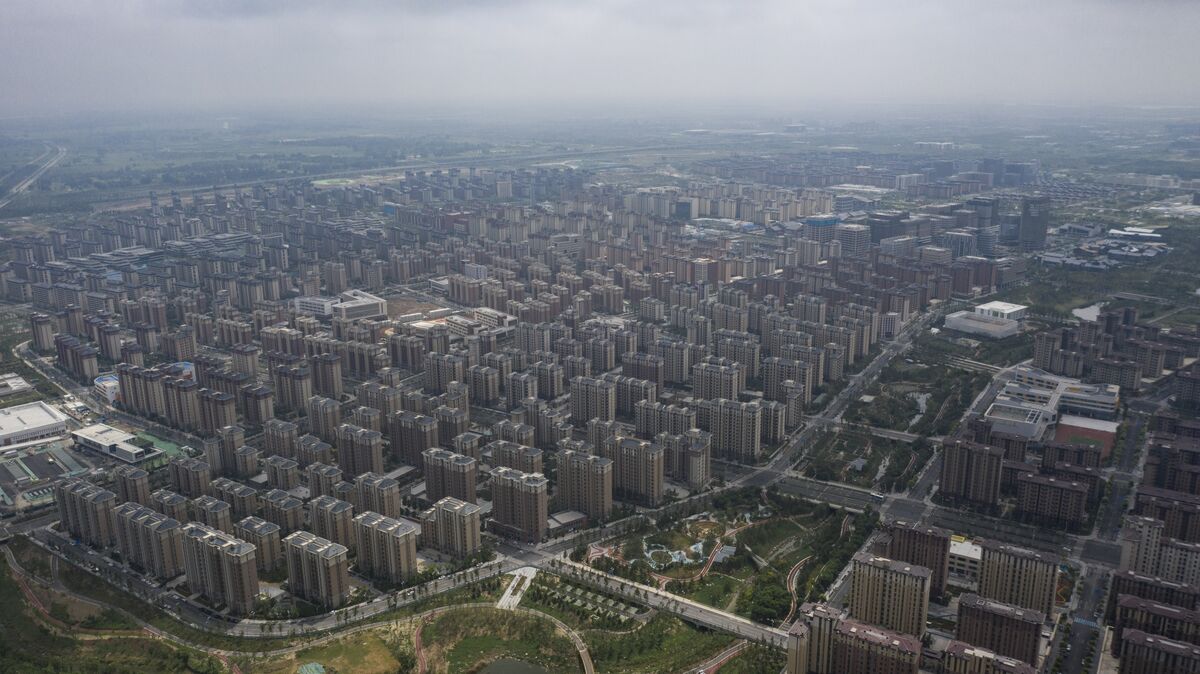This aerial photograph captures a sprawling cityscape dominated by densely packed high-rise buildings, their uniformity suggesting they are residential apartment blocks. The overwhelming color palette of the image is a monotonous brown, as nearly all the structures share this hue. The top-down view reveals a heavily industrial and uninviting environment, accentuated by a persistent smog that casts a grayish tint over the scene, obscuring the sky and adding to the overall drab atmosphere. Towards the bottom of the image, there is a noticeable splash of green indicating a park area that starts at the bottom left and stretches upwards towards the right, providing a stark contrast to the otherwise concrete expanse. This greenery, however, does little to alleviate the overwhelming sense of congestion and bleakness. The location is not specified, but the image evokes thoughts of densely populated regions in East Asia, such as China, Japan, or even areas reminiscent of North Korea, and possibly European or Russian cities known for their extensive urban sprawl. The absence of natural elements like birds and visible sunlight further underscores the stark, urban character of this vast and closely built environment.